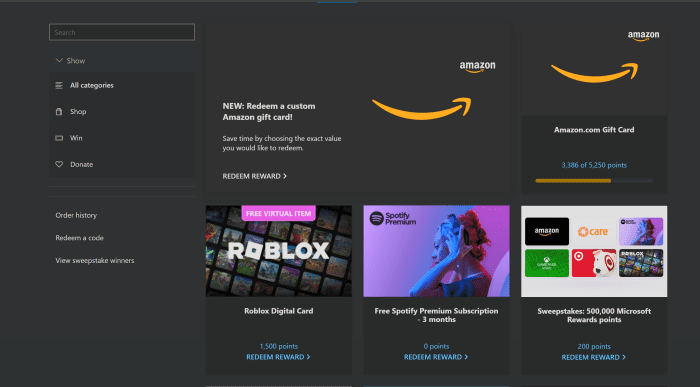The image showcases a section of Amazon's website against a sleek black or charcoal gray background. In the upper right corner, the distinctive Amazon logo is prominently displayed, accompanied by a few of Amazon's signature swooshes scattered across the backdrop. On the far left of the image, a vertical menu presents a series of navigation options.

At the top of this menu, there is a search box labeled "Show" with a down arrow, indicating a dropdown menu that likely offers filter options such as "All Categories," "Shop," "Win," or "Donate." A new feature is highlighted—the ability to redeem a custom Amazon gift card. Users are encouraged to save time by selecting the exact value they wish to redeem. Below this, a variety of rewards are listed, showcasing different redemption options:

- **Roblox Digital Card:** Available for 1,500 points, users can redeem this reward for a digital card suitable for Roblox.
- **Spotify Premium Subscription:** Offers a free three-month Spotify Premium subscription as a redeemable reward.
- **Microsoft Rewards Sweepstakes:** Users can enter a sweepstakes to win 500,000 Microsoft reward points by redeeming this option.

The layout and options suggest an enticing system designed to attract users into redeeming rewards, which could potentially draw them into services such as Roblox and Spotify.